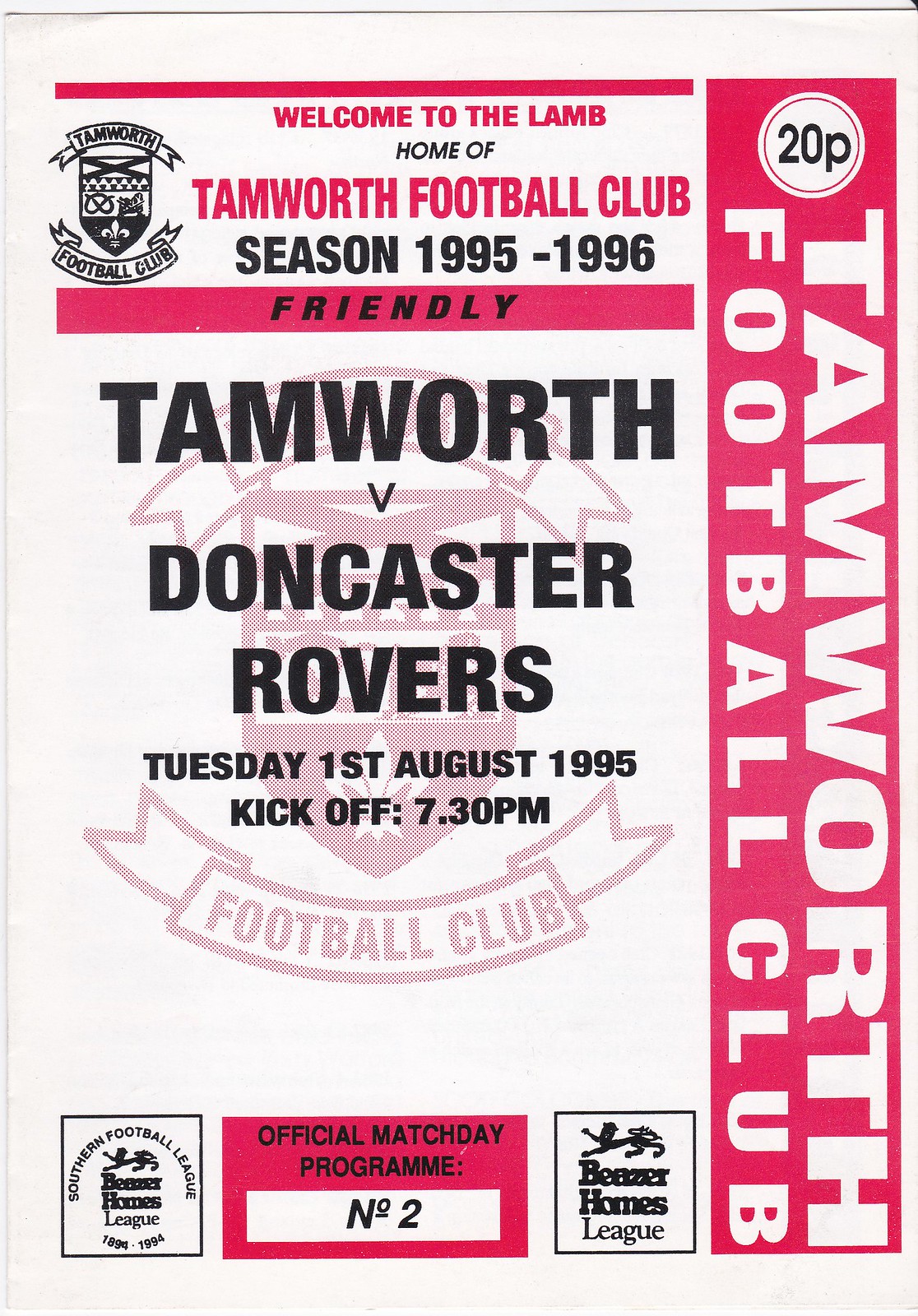This is a color image of a football program cover, prominently featuring a white background with pink bars and text, with the majority of the writing in black. At the top, in pink, it reads "Welcome to the Lamb, Home of Tamworth Football Club," while in black, it states "Season 1995-1996, 20p." Running vertically on the right-hand side, in pink and white, is the text "Tamworth Football Club." The center of the cover highlights the match details in black letters on a white background: "Tamworth v. Doncaster Rovers, Tuesday 1st August 1995, Kickoff 7.30pm." At the bottom, it is noted as "Official Match Day Program Number 2." The design is primarily text-based with the club's name positioned vertically in an angled layout on the right and the match details centrally aligned, embodying a clean and straightforward printed press style.